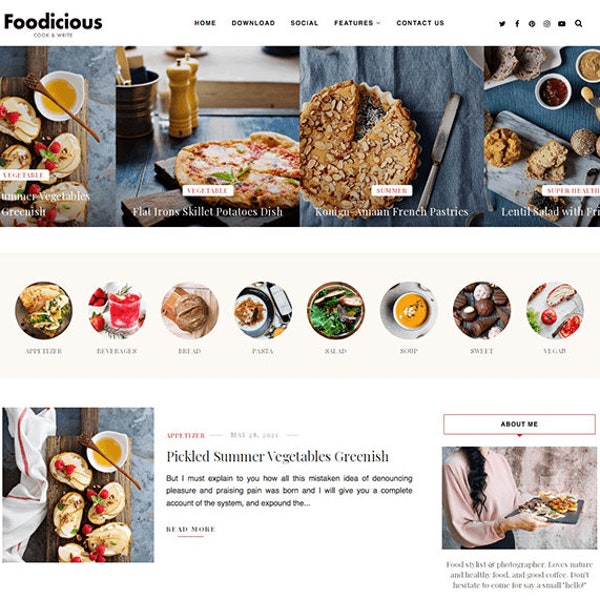Screenshot of a food-themed website showcasing a variety of dishes. The website features a vibrant layout with high-quality images of several enticing meals, including a flat iron-grilled skillet potato dish and a pie, among others. The dishes are presented in red, circular image thumbnails against a gray background. A highlighted section at the bottom of the page, with a greenish rectangular image, advertises "Pickled Summer Vegetables." 

The website includes an "About Me" section with detailed information about the blogger or website owner. The top navigation bar is displayed in bold, black, uppercase text with links to sections such as Home, Download, Social, Features, and Contact Us. Social media logos for Twitter, Facebook, YouTube, and Instagram, along with a search icon, are located in the top-right corner, all in black. The website features a clean, white background that helps make the colorful food images stand out.